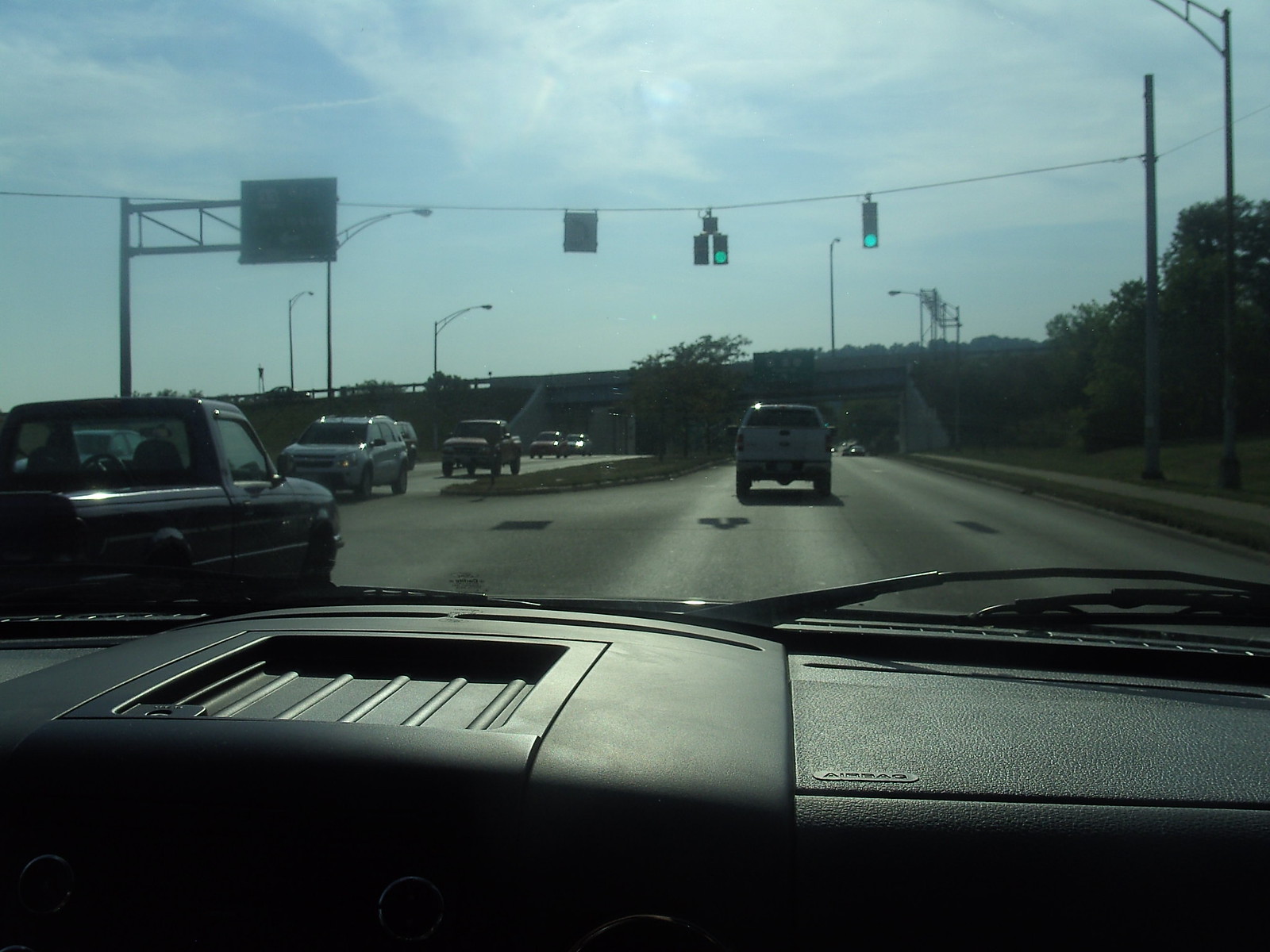This photograph captures a dynamic street scene viewed from inside a car, looking out through the front windshield. Despite the bright sunlight of the day, the lighting in the image appears slightly dim. Inside the car, the dashboard is visible, and the windshield wipers rest in their down position, indicating a dry, sunny day. 

Ahead, a car several lengths in front is passing through a green traffic light. In the adjacent left lane, another vehicle is slightly further ahead, also preparing to move through the green light. On the opposite side of a grassy median, vehicles can be seen traveling in the opposite direction.

To the right of the scene, a guardrail runs alongside a dense stand of trees, providing a natural backdrop. Up ahead, more trees line the roadside, and the vehicle is approaching an overpass, which sits a few yards beyond the traffic light. The image captures the essence of a typical drive on a sunny day, with a mix of natural and urban elements converging.